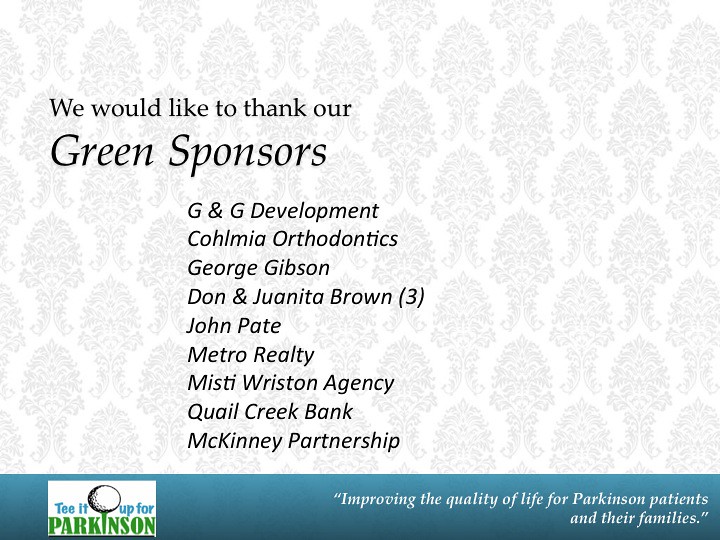The image appears to be an advertisement with a white background and a subtle gray floral spade pattern. Dominating the left-hand center of the image, in black text, it expresses gratitude with the words: "We would like to thank our Green Sponsors," where "Green Sponsors" is prominently sized. Listed below are the sponsors: G&G Development, Colmia Orthodontics, George Gibson, Don and Juanita Brown, John Pate, Metro Realty, Misty Wriston Agency, Quail Creek Bank, and McKinney Partnership, with a peculiar "(3)" beside the Browns. At the bottom, a blue horizontal stripe extends across the image. Within the stripe on the bottom left, a white square contains the text: "Tee it up for Parkinson's," where "Parkinson's" is in bold green with the "I" cleverly designed as a golf tee holding a ball. Meanwhile, on the bottom right in white lettering, the message reads: "Improving the quality of life for Parkinson's patients and their families."